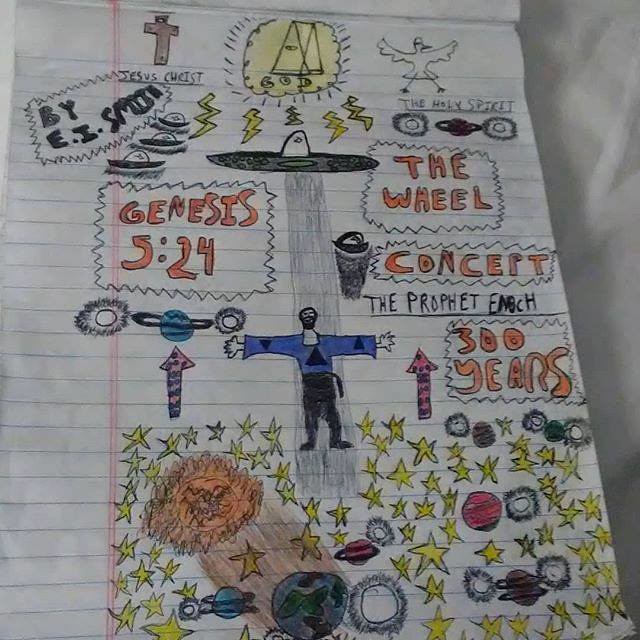This image showcases a vibrant doodling and sketching session on notebook paper. The artist has employed a combination of colored pencils and markers to create an eye-catching array of celestial motifs. At the bottom of the page, a series of yellow stars adds a luminous touch. A variety of planets populate the scene, including a red Saturn-like planet with a distinctive ring, a classic Earth depicted in blue and green, and additional Saturn-inspired planets colored in brown and blue, each with unique ring patterns. 

Adding to the cosmic theme are several suns, rendered in black and white, their uncolored forms suggesting an imaginative flexibility. Embedded within the artwork are textual elements, including a Bible verse, "Genesis 5:24," and two inscriptions titled "The Wheel" and "Concert," the latter in striking orange. The notebook page is filled with an eclectic mix of doodles, capturing a sense of creative exploration and boundless imagination.